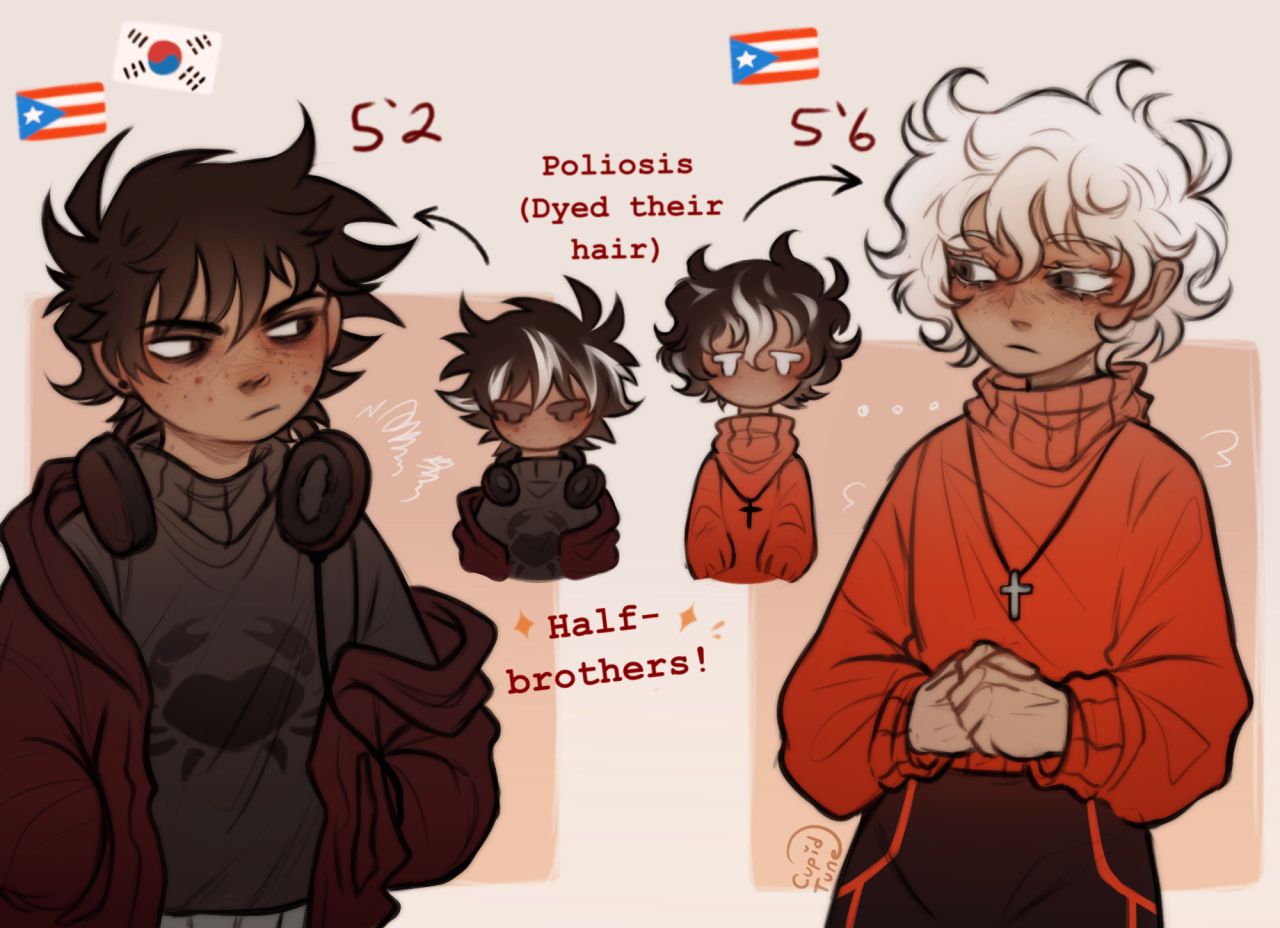This vibrant, landscape-oriented anime graphic presents a detailed digital illustration, possibly intended for a webtoon or fan art. It depicts two half-brothers, their relationship emphasized by the caption, "half-brothers." The left figure, standing at 5'2", sports wild black hair, brown skin, and an emo-goth aesthetic with black headphones, a black sweatshirt, and a maroon jacket. His doubtful expression contrasts with his attire. The right figure is taller at 5'6" with white curly hair, a red long-sleeve sweater, and a religious cross necklace. He also has darker skin and gazes down at his brother with a frown. Both figures display unique cultural backgrounds: the left adorned with a flag showcasing a red and blue yin-yang symbol, and the right with a flag bearing red and white stripes and a blue pennant with a white star. In the center of the image, smaller versions of these characters are annotated with notes, including "Poliosis (dyed their hair)" and "half-brothers!" The intricate detailing hints at deeper character backgrounds, making the illustration intricate and engaging. The artwork title, "Cupid Toon," is noted at the bottom, potentially hinting at the series or artist's name.